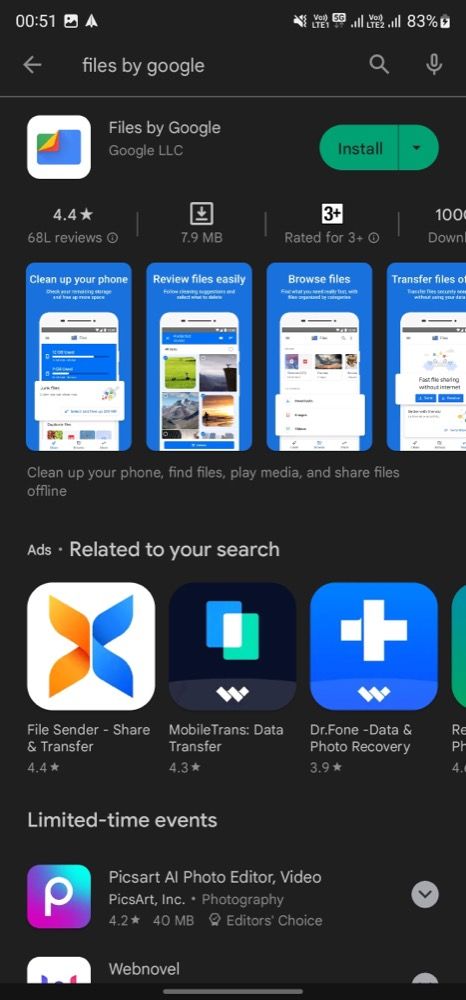**Caption:**

The image depicts a smartphone screen captured at 00:51. The screen shows an app information page from the Google Play Store displaying the "Files by Google" application. Key icons and elements are present, including a picture icon, a triangle play button indicating no sound, a volume control, brightness level, signal strength bars, and an 83% battery charge indicator.

At the top of the screen, a left arrow icon is visible next to the app name "Files by Google," followed by a search icon and a microphone icon. Beneath this row is a horizontal line separating the header from the primary content.

The information presented includes:

- **App Name**: Files by Google
- **Developer**: Google LLC
- **Action Button**: Install (green dropdown button)

Additional details about the app are provided:

- **Description**: Clean up your phone
- **Rating**: 4.4 stars based on 68 reviews
- **Download Size**: 7.9 MB
- **Age Rating**: Rated for ages 3+
- **Downloads**: 100 million (partially cut off in the text)

The summary of features includes cleaning up your phone, finding files, playing media, and sharing files offline.

Below the app description is an ad section related to the user's search, featuring the following apps:

- **File Sender**: Share and Transfer - 4.4 stars
- **Mobile Trans**: Data Transfer - 4.3 stars
- **Doctor Phone**: Data and Photo Recovery - 3.9 stars
- **Limited Time Events**: PicsArtArt

This comprehensive view gives detailed insights into the "Files by Google" app and related applications available for download.